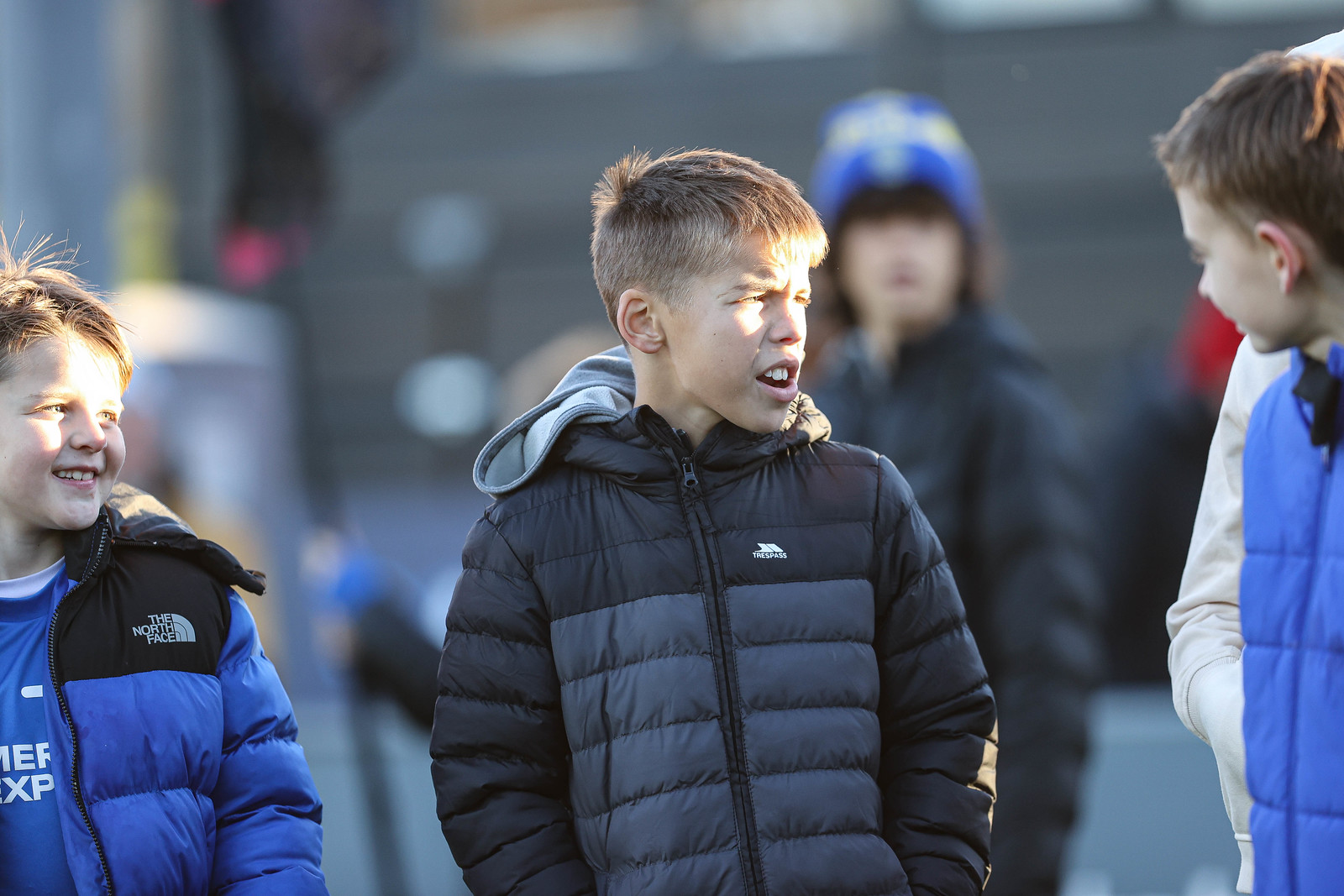The photograph captures a candid moment of three middle school-aged boys, each dressed in puffy winter jackets, engaged in what appears to be a lively conversation. The boy in the center, with short light brown hair combed forward, wears a black and gray puffy jacket, zipped all the way up, and a gray hoodie with a white emblem peeking out. His head is turned to the left, squinting slightly, with his lips parted as if speaking or reacting in surprise. To his right, our left, stands a shorter boy, smiling and looking up at him; he's dressed in a blue and black North Face jacket with sunlight softly illuminating his forehead. On his left, our right, is another boy in a blue puffy jacket, slightly out of focus, turning his head towards the center boy with a hint of redness on his ear. In the background, a woman, also out of focus and wearing a blue and white beanie and a dark jacket, silently observes the scene. The sun casts a gentle glow on parts of the boys' faces, suggesting they might be outside, either on a street or at a playground, sharing a lighthearted moment.